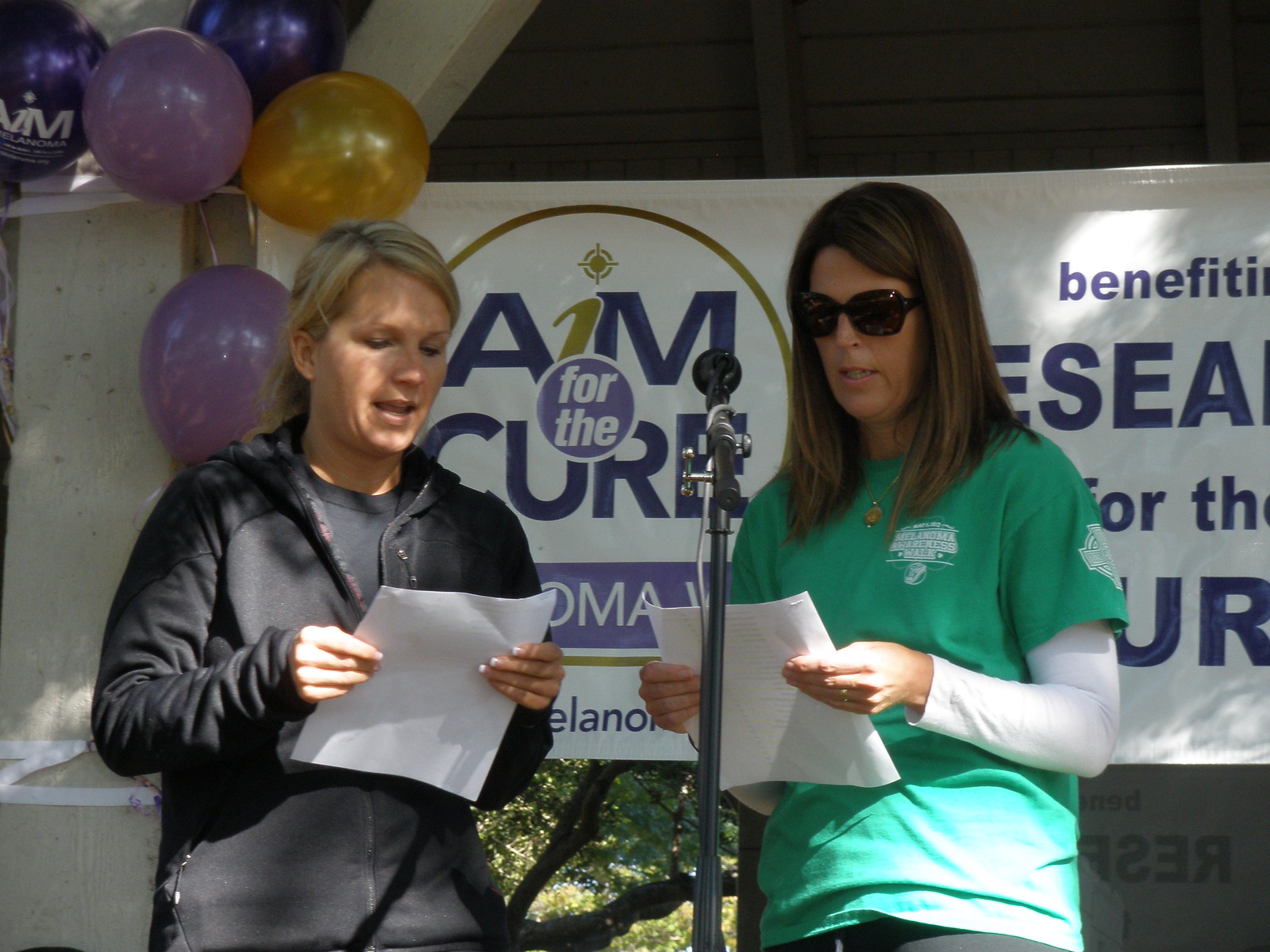In this outdoor photograph taken on a sunny day, two women are standing on a stage, evidently participating in a charity event. The stage is adorned with a white banner that reads, in purple font, "Aim for the Cure," along with partly obscured text mentioning it benefits research. Behind them, a mix of vibrant balloons in purple, gold, and black accentuates the setting.

The woman on the left has blonde hair and is dressed in a black sweatshirt over a black t-shirt. She holds a white piece of paper in her hands, seemingly reading from it. Next to her, the woman on the right, with shoulder-length brunette hair and large dark sunglasses, stands in front of a black microphone. She is clad in a green t-shirt with white long sleeves beneath, paired with black pants. She's also holding a white piece of paper, from which she appears to be reading.

The background features a large tree with lush green leaves, and there's visible grass and bushes indicating the stage is set in a park or a similar outdoor environment. The bright daylight filtering through the scene underlines the daytime setting.